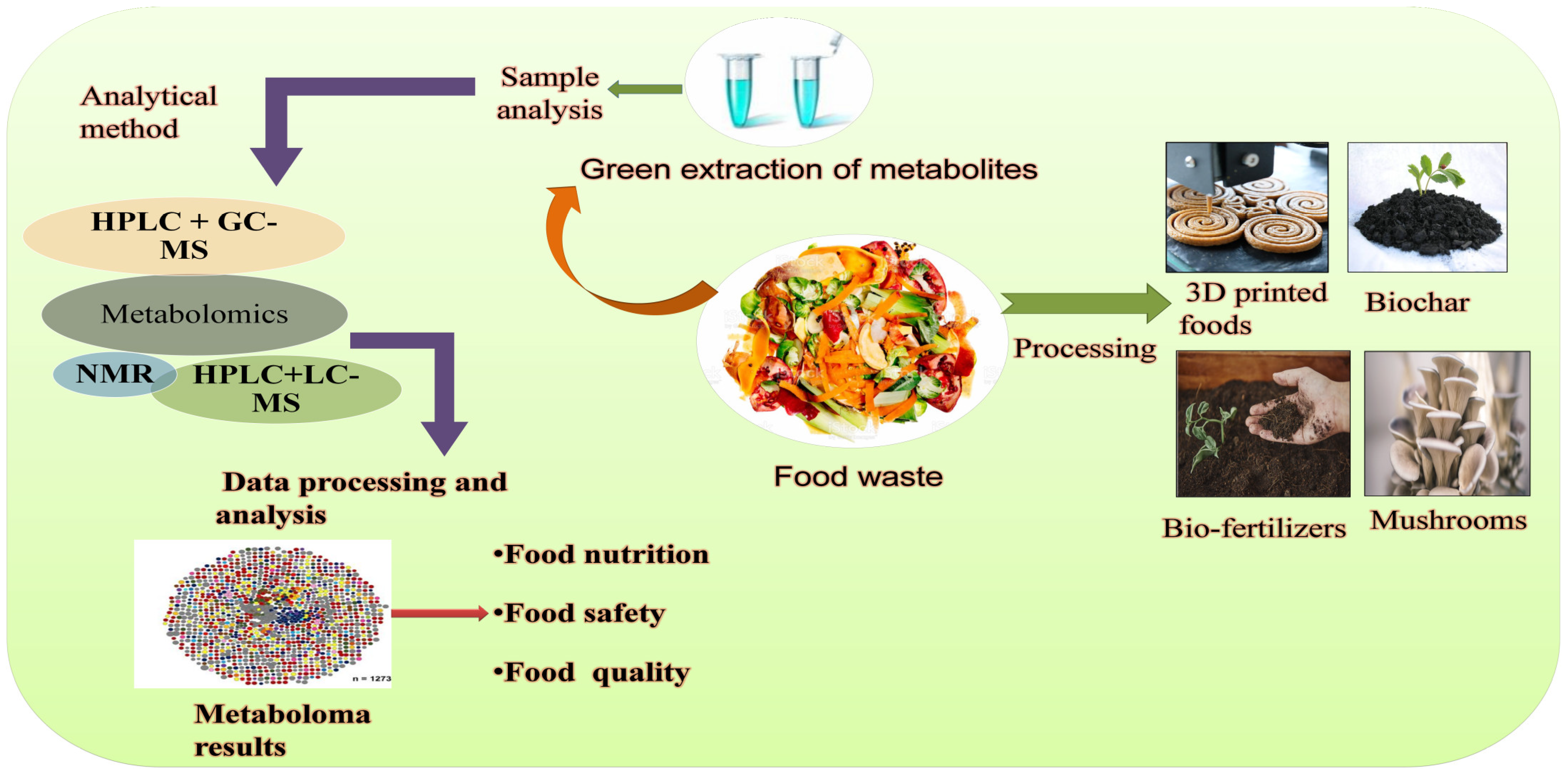This detailed square infographic, set against a subdued lime-green background, presents a comprehensive flowchart related to food waste and metabolomics. At the top center, two beakers containing blue liquid mark the starting point labeled "Sample Analysis." An arrow extends leftward and then curves downward to "Analytical Method." From there, the chart progresses through a series of oval shapes with black scientific writing, reaching "Metabolomics." Another arrow directs downward toward "Data Processing and Analysis," leading to a circular shape filled with rainbow-colored circles and labeled "Metaboloma Results."

Continuing, the flowchart identifies three key areas: "Food Nutrition," "Food Safety," and "Food Quality," with "Food Waste" being prominently displayed in the middle. Moving rightward from "Food Waste," the chart illustrates various processing outcomes, pointing towards potential products like "3D-Printed Foods," "Biochar," "Biofertilizers," and "Mushrooms." Additionally, an arrow curves upward from "Food Waste" to "Green Extraction of Metabolites," again reinforcing the chart's cyclical focus on sustainable practices and innovations in food processing and safety. A central image of a plate filled with salad-like food visually anchors the concepts presented.